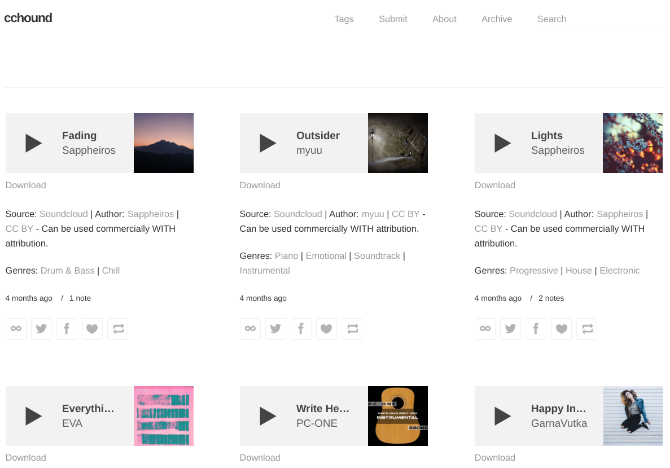This image showcases a webpage titled "Seahound," prominently displayed at the top with several navigational tabs, including "Tags," "Submit," "About," "Archive," and "Search." Below these tabs is a curated collection of images and song listings.

The first entry is titled "Baiting" by Sapphire Heroes, accompanied by an evocative image of a mountain at sunset. The listing includes a play button and a download option, with the source indicated as SoundCloud. The track's genre is specified as drum and bass, chill, and it was uploaded four months ago.

Following this, the next song is "Outsider" by Mayu. This entry includes a download button and mentions SoundCloud as the source. The genres are tagged as piano, emotional soundtrack, and instrumental.

Next, the song "Lights" by Sapphire Heroes is featured. This track is also sourced from SoundCloud, with Sapphire Heroes credited as the artist. The listing specifies that it can be used commercially with attribution. The genres include progressive, house, and electronic.

The fourth listing is for the song "Everything" by Eva, which features a pink and green album cover. This entry includes both a black play button and a download button.

Following this is a partially visible title "Righty," featuring an image of a round guitar on a black background.

The final song listed is "Happy Inn" by Gamma Vutka, which includes an image of a person jumping high in a sleek outfit.

The overall design of the page includes a white background with black text, and play buttons are provided for each song to facilitate instant listening.